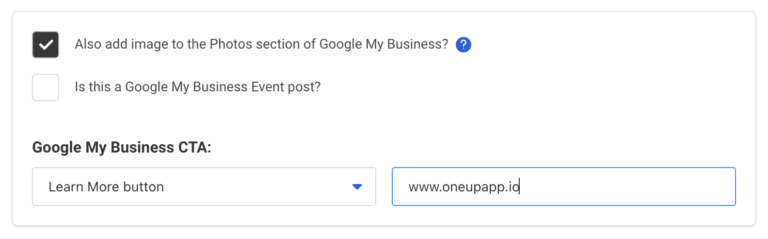The image displays a user interface with various elements related to Google My Business. On the left side, there are two smaller squares. The top square is black with a white checkmark and contains the prompt, "Also add image to the photo section of Google My Business?" accompanied by a blue circle with a white question mark inside it. The square beneath it is unchecked and asks, "Is this a Google My Business event post?"

Below these options, in bold text, is the label "Google My Business CTA." To its right, there's an elongated white box with the text "learn more button." Adjacent to the white box, there appears to be a downward-facing blue toggle, suggesting the option to click for more choices.

Further to the right, there is an active blue text box where someone is typing a website address. The URL entered is "www.oneupapp.io," although the text is displayed as "www.1upap.io," indicating that the user might still be in the process of typing. The highlighted box likely indicates that it is currently being edited.

The background of the image is white, providing a clean and uncluttered appearance. There are no additional elements present in the image.